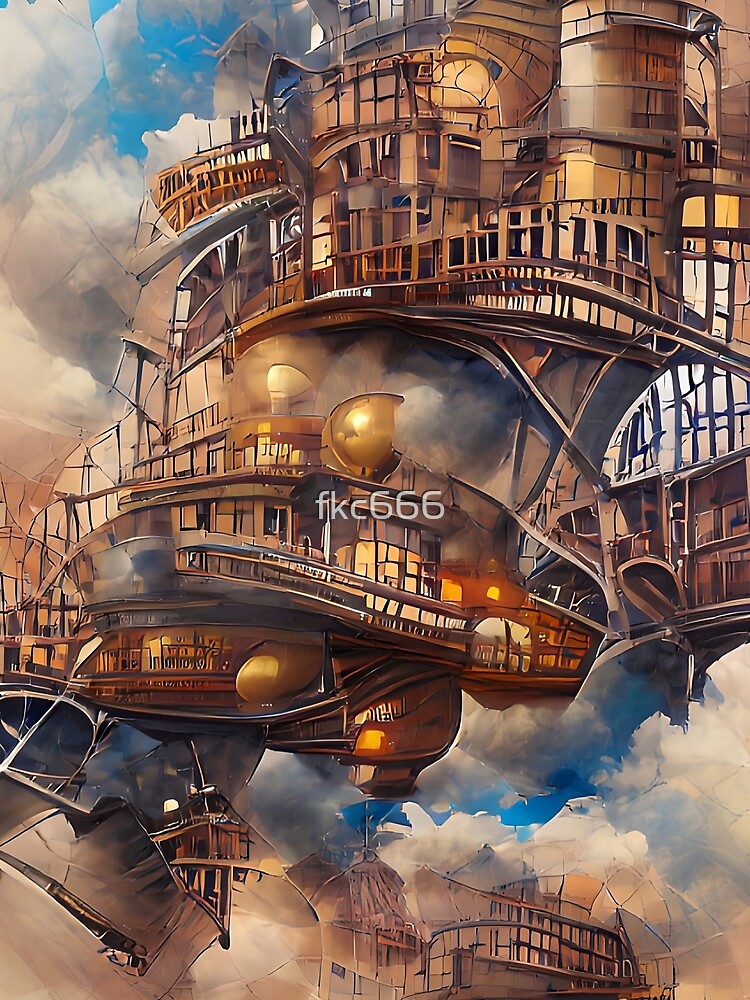The image depicts a highly detailed, abstract, and multi-colored artistic creation, evoking an otherworldly dream city. The scene features a complex, brown structure that rises and falls with multi-level walkways, decks, and variously sized windows. Spiraling curves and an intricate, tower-like design dominate the composition. Surrounding the structure is a vibrant sky filled with clouds, both above and below, lending a surreal, almost floating appearance. In the center of the image, a white watermark with the lowercase letters "fkc" and the number "666" stands out against the background. The entire piece lacks a definitive border or background, immersing the viewer in its surreal and dreamlike context. While some elements hint at architectural features, such as streets, towers, and orbs, the true nature of the vessel or city remains an enigma, firmly rooted in the realm of imagination and artistic expression.